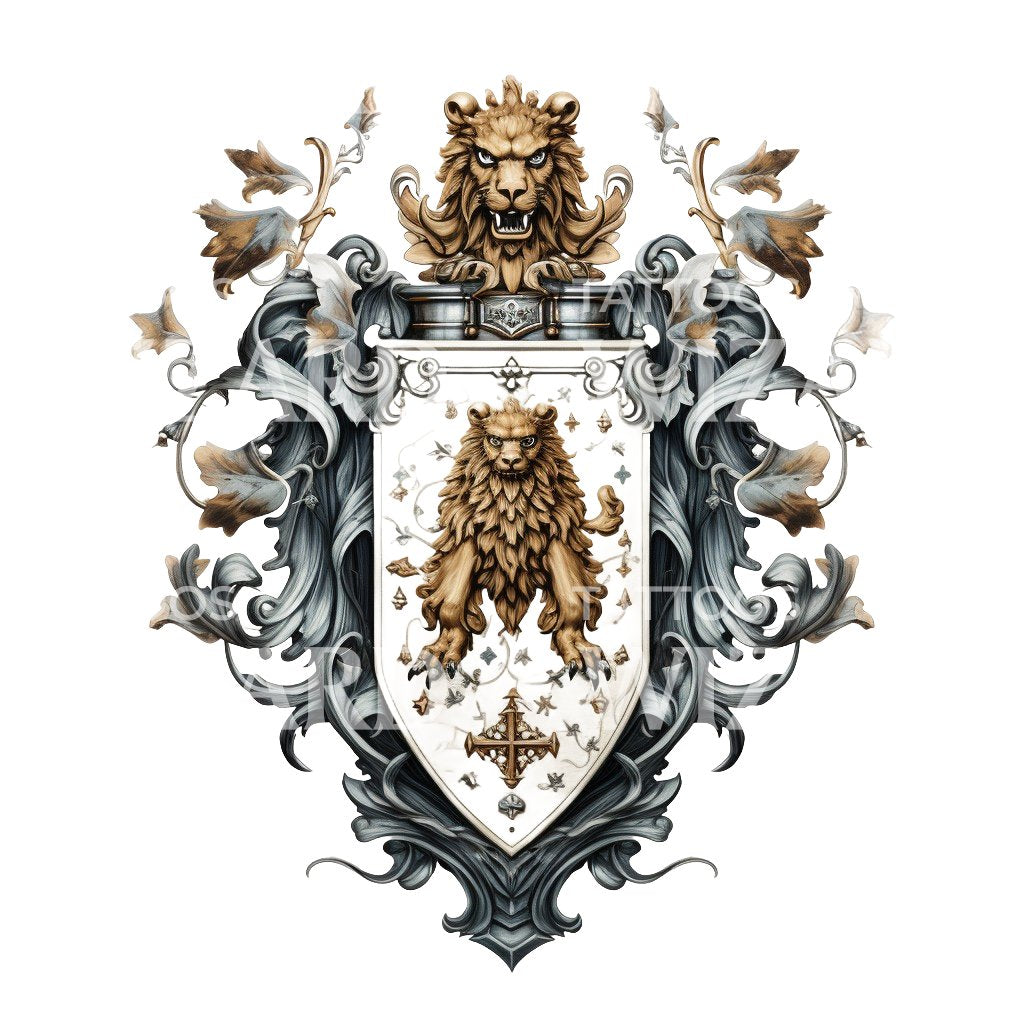The image depicts a detailed, computer-generated royal crest, rich in medieval heraldic elements. At the top of the crest is a fierce-looking lion's head, drawn with a gold hue, its mouth open revealing sharp white teeth. Below this lion's head is a large, ornate shield which features a smaller, inner shield at its center. The main shield is adorned with intricate grayscale filigrees, including leaves, vines, and abstract patterns resembling flowing silver waves, with some areas exhibiting plaid stripes. The inner shield, set against a solid white background, houses a fantastical griffin-like creature, combining the characteristics of a lion and an eagle. This mythological creature, like the lion head above, is rendered in a matching gold color and stands above a gold cross, emphasizing its regal and mythical nature.